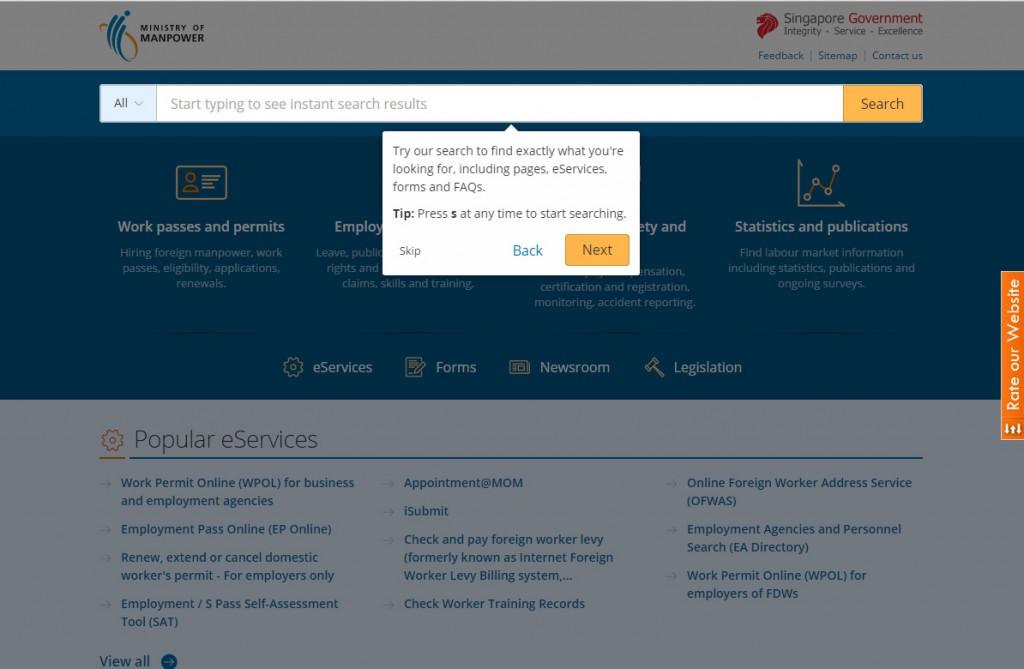This cropped desktop screenshot captures the homepage of the Singapore Government's Ministry of Manpower website. The header is predominantly white, featuring the Ministry of Manpower logo on the top left, accompanied by the Singapore Government logo to its right. Below these logos, a phrase—'Integrity Service Excellence'—is elegantly inscribed in small grey letters. 

Beneath the header, three navigational categories—Feedback, Sitemap, and Contact Us—are aligned on the top right. Centrally located below this is a large search bar designed for ease of access. The search bar includes a dropdown box on its left side, set to "All" by default, offering a comprehensive search across various categories. The placeholder text inside the search bar reads, "start typing to see instant search results," in a grey, user-friendly font. 

An active search interaction is depicted, with an orange-highlighted search bar prompting a pop-up message underneath. This message encourages users to "try our search to find exactly what you're looking for, including pages, e-services, forms, and facts." Additionally, a tip on initiating a search by pressing 'S' at any time is provided on the right side of the search bar.

The pop-up interface further includes navigation options, with 'skip' in small black letters on the bottom left and 'back' in blue letters on the bottom right. A prominent orange "next" button is also visible on the far bottom right, inviting users to proceed with their search journey.